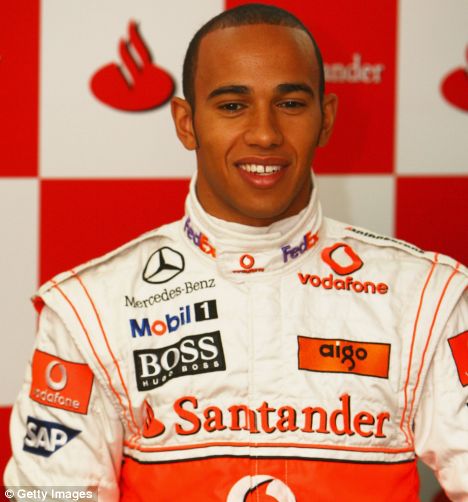This is a detailed photograph showcasing a race car driver, captured from the lower chest to the top of the head. The image prominently features the driver's race suit, which is meticulously zipped up. The suit's design blends a white top half and sleeves with an orange bottom half while incorporating striking orange stripes on the shoulders. Various sponsor logos adorn the suit, adding a lively mosaic of brand identities. On the left sleeve, an orange rectangle prominently displays "Vodafone" in white text, complemented by a large circle logo above it. Directly below, another logo shows "SAP" in white text. Other logos scattered across the chest and arms include well-known brands such as Mercedes-Benz, Mobil 1, Boss, Hugo Boss, Santander, Igo, Vodafone, and FedEx.

In the backdrop, blurred red and white checkerboard patterns suggest an association with sponsorship or event branding typical in the racing environment, though the specific text is indistinct. Additionally, there is a watermark in the bottom left corner imposed over the photograph, consisting of a see-through black rectangle with white text that reads "copyright Getty Images." The driver, assumed to be younger, stands poised and ready, epitomizing the essence of competitive racing.